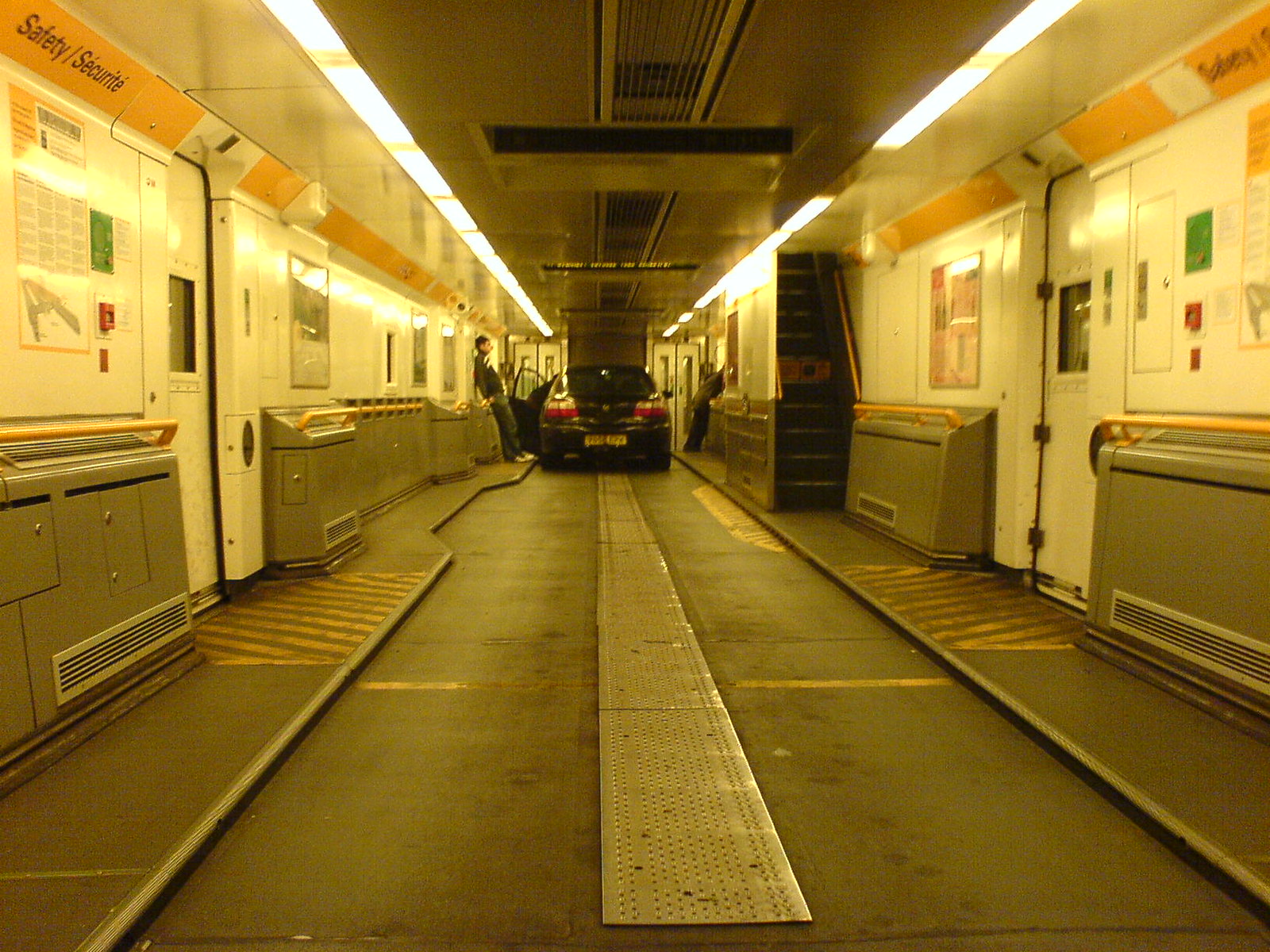The photograph depicts the interior of what appears to be a repair shop or a ferry designed to move cars. The setting resembles a tunnel with a roof featuring grates along the ceiling for ventilation, illuminated by fluorescent track lighting that emits a yellow, murky glow. The word "SAFETY" is prominently displayed across the ceiling. The floor is made of grey concrete and prominently features a long, shiny metal track running its entire length, which is mirrored by a similar but less shiny metal piece on the ceiling filled with ventilation holes.

The walls are a combination of white and grey, with doors and windows potentially leading into other parts of the building. Toward the back of the image, a black car with a partially opened driver's side door is visible. A person is seen leaning against the wall near the car, and multiple people can be seen further up, giving the space an active, bustling atmosphere. The car has distinct red and white light fixtures and a yellowish license plate. One of the lighting bulbs on the ceiling’s right side is out, adding to the functional yet work-in-progress ambiance of the place.